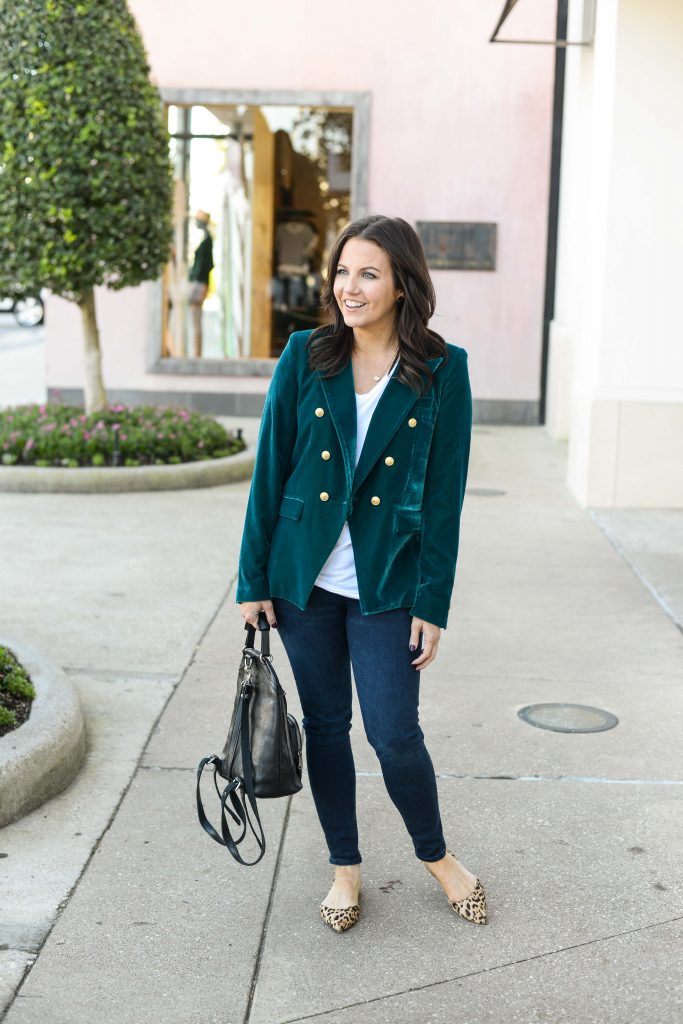This is a photograph of a Caucasian woman, probably in her 20s, standing in an outdoor shopping area in front of a sophisticated-looking store with mannequins displayed in the window. She is holding a black backpack purse by its handle in her right hand, with the backpack straps hanging down. The woman is dressed stylishly in tight dark blue jeans that reach her ankles and leopard print ballerina flats. She wears a white top underneath a green velvet double-breasted blazer adorned with gold buttons. Her medium-length brown hair is parted down the middle, and she is accessorized with a gold necklace and dark nail polish. The woman has a bright smile on her face, as if she has just noticed something surprising or familiar to her right. In the background, there is a circular cropped tree positioned on the concrete ground, enhancing the upscale, outdoor shopping environment reminiscent of a Beverly Hills shopping center.